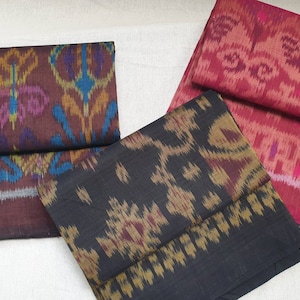This photograph showcases three different fabric swatches, each marked by distinct tribal and Aztec-inspired patterns, spread over a light gray background. 

In the upper left corner, there is a dark brown to maroon fabric adorned with intricate designs featuring red flowers, blue and orange elements, and a prominent helmet-like motif with a yellow border around a red interior. 

The bottom fabric in the foreground is predominantly black with yellow and red snowflake-like patterns, along with vine-like motifs. Notably, within this print, there appears to be an abstract shape resembling a mouth with an eyeball. 

On the right side, a pink cloth features lighter pink designs and dark red accents. Additionally, there are a few visible letters, hinting at the word "patrol," partly concealed under the black fabric. 

Each swatch is folded over, emphasizing their individual textures and vibrant, complex designs.